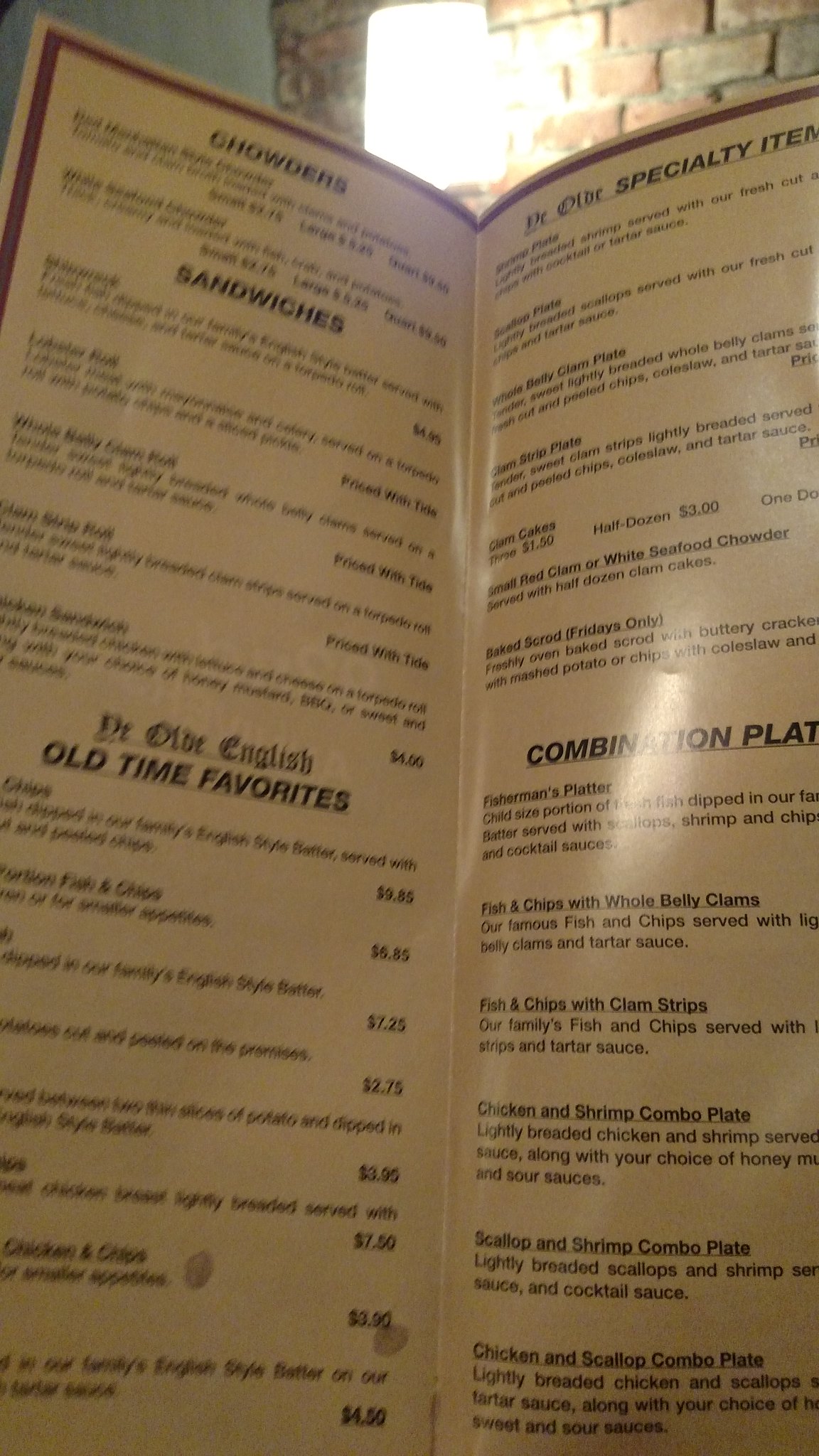The image captures an open menu positioned slightly at a distance, allowing partial readability of the bold text. A square yellow light fixture at the top of the photo emits a bright white light, illuminating a brick wall backdrop, with a hint of a blue wall on the left side. The menu itself is beige with a maroon outline, prominently displaying various sections in bold black text. 

The first section, labeled "Chowders," features about four lines of smaller text beneath the heading. Further down, the section titled "Sandwiches" lists five different options under its bold heading. Below this, in cursive script, the menu reads "The Old English," followed by a section termed "Old Time Favorites," featuring several dish names accompanied by prices. 

In the upper-right corner of the menu, the label "Specialty Steak" or "Specialty Item" can be discerned, listing specific choices underneath. Finally, at the bottom, the word "Combination" appears, partially obscured, with "P-L-A-T," which likely abbreviates "Combination Platters."